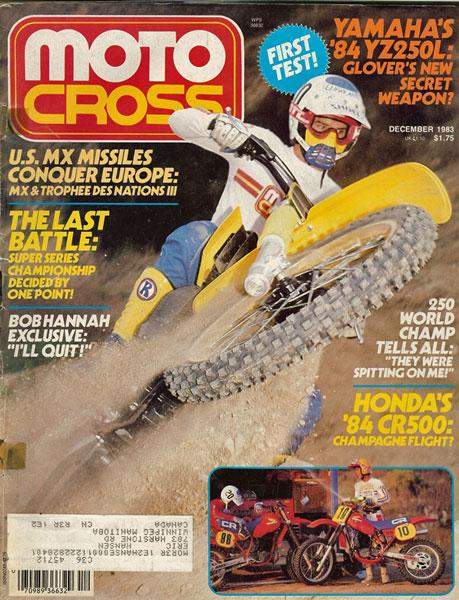This is the cover of an old edition of Motocross Magazine from December 1983, priced at $1.75. The prominent title, "Motocross," is displayed in a bold red and yellow logo at the top. The upper right corner features a headline about "Yamaha's '84 YZ250L, Glover's new secret weapon," accompanied by the caption, "250 world champ tells it all, they were spitting on me," and a mention of Honda's '84 CR500 described as a "champagne flight?"

The central image captures an action shot of a motocross rider, dressed in a white top and red goggles, intensely navigating a turn with dirt dramatically kicked up from the front wheel. The motorbike, which appears to be yellow, adds to the dynamic feel of the scene. 

Additional details populate the cover: the lower right corner boasts a smaller photo of two other riders, bringing more action elements into the composition. Text along the bottom and edges highlights major articles, including "Last Battle Super Series Championship decided by one point," and a Bob Hanna exclusive with the quote, "I'll quit." The cover is completed with a barcode and an upside-down mailing label in the bottom left corner, reinforcing its vintage, well-read nature.